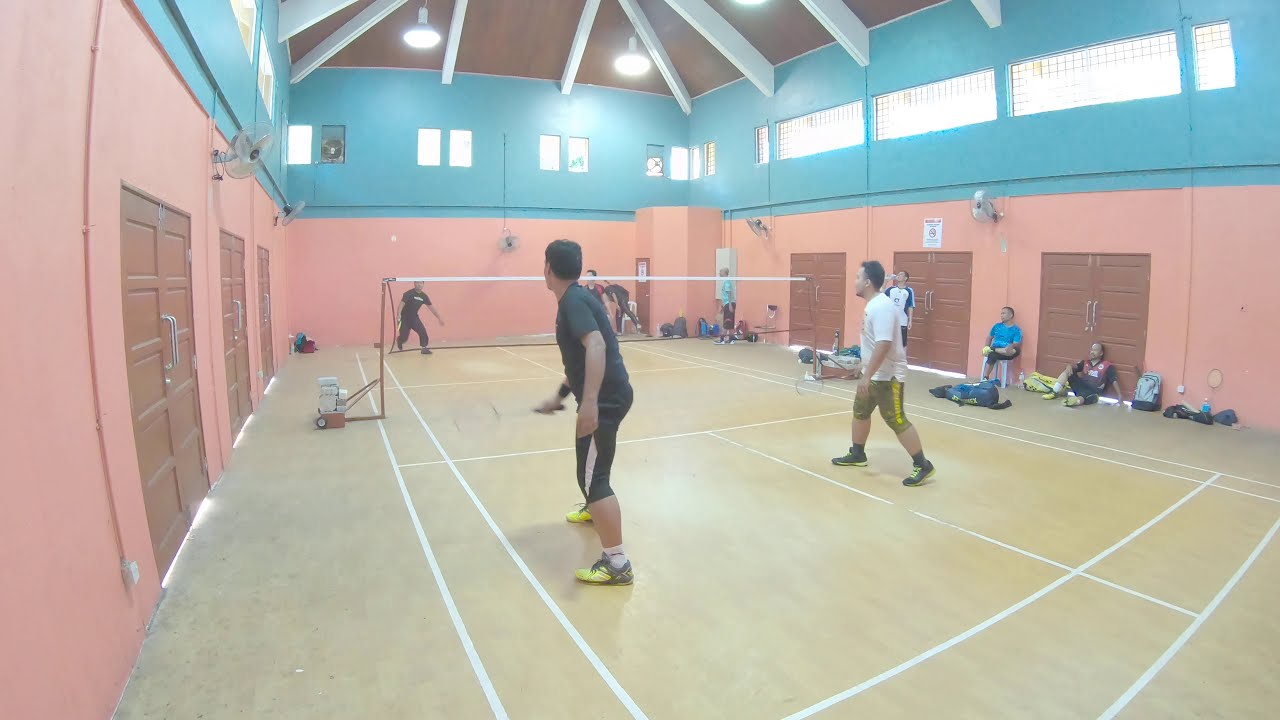In this detailed image, we see an indoor gymnasium with a court where four men are playing doubles badminton. The court's floor is a light-colored hardwood with white lines marking the boundaries. The walls have a two-tone color scheme: light blue on the upper section and pink on the lower section where the doors are located. There are two sets of three double dark brown doors on each side of the court, each with large silver handles in the center. Above these doors are wide rectangular windows. At the back, a thinner door has a white poster affixed to it, flanked by vertical windows.

On the court, each player stands in their designated boxes with a net separating them. Closest to the camera, the player on the left wears a black t-shirt and black shorts with white stripes. His partner, on the right, is dressed in a white t-shirt, tan shorts with yellow stripes, and black tennis shoes. Opposing them, the player on the left wears a black t-shirt and black sweatpants, while his teammate on the right sports a black t-shirt with red stripes on the sleeves. 

In addition to the players, there are several people standing or sitting along the right wall, some with backpacks and bags, likely spectators watching the game. This detailed snapshot captures the competitive spirit and the environment of an indoor badminton match.